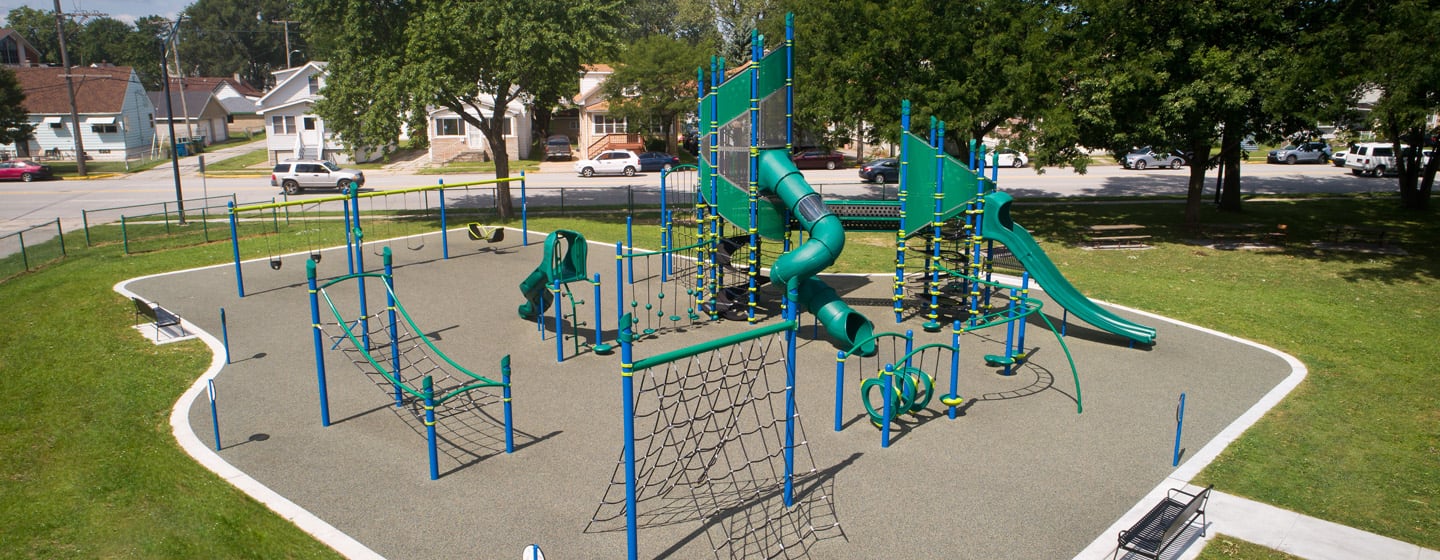The photograph, taken outdoors on a sunny day from an elevated position, captures a horizontally rectangular scene dominated by a vibrant, green neighborhood park. The backdrop of the image features a row of lush, deciduous trees lining a residential street, with middle-class houses and a few parked cars, including SUVs.

In the foreground, the fenced-off park is the focal point. The playground within boasts a variety of equipment set against a gray surface bordered by cement. Among the playful structures are multiple slides, including a straight one and a couple of twisty ones, as well as rope ladders and nets resembling accessible army drills. Swing sets are also prominently featured.

For the comfort of visitors, the park includes several black benches, strategically placed on both the right and left sides. Additionally, there's a mention of lighting, indicating that the park is suitable for evening play as well. The overall scene is a lively and inviting depiction of a well-utilized community space.